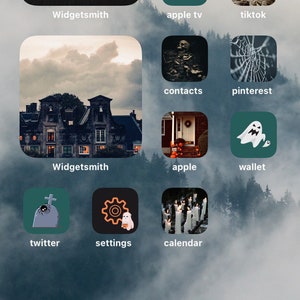The image appears to be a zoomed-in view of a smartphone home screen featuring a Halloween-themed wallpaper and several app icons. The background showcases a dark, atmospheric forest shrouded in thick white fog, with dark green trees barely visible through the mist. As for the app icons, the first three at the top are partially cut off, displaying white sections.

Along the left side, the app arrangement includes:
- "Widget Smith" at the top with a dark, indiscernible background.
- "Apple TV" beneath it, paired with a green-tinted background.
- "TikTok," set against a beige or brown backdrop.

A larger widget labeled "Widget Smith" spans the length of two rows, depicting a spooky house with lights on, surrounded by a cloudy sky.

On the right side of the screen, the row of apps is as follows:
- "Contacts" with an icon featuring skeletons.
- "Pinterest" with a spider web-themed icon.
- "Apple" accompanied by an icon of jack-o'-lanterns lining the stairs to the house.

At the bottom row, the apps include:
- "Wallet" with an icon showing a white ghost chasing a smaller white ghost.
- "Twitter" featuring a tombstone with a spider.
- "Settings" represented by a gear icon with a ghost.
- "Calendar" with an icon that includes several lit white and gray candles.

The overall theme is decidedly eerie, aligned with Halloween motifs and emphasizing a spooky, mist-filled forest setting.